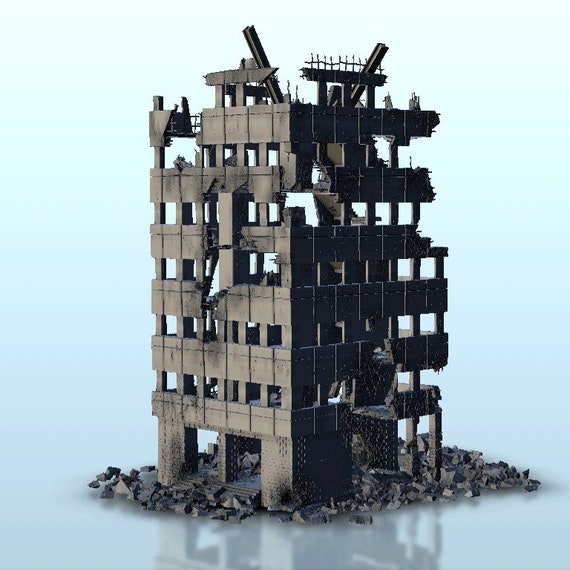This detailed caption blends the input from all three descriptions into a cohesive narrative:

"This image depicts a derelict, partially collapsed skyscraper, likely a computer-generated representation. The eight-story concrete structure, devoid of windows and doors, sits on a light blue, slightly reflective surface, which transitions into a pale blue and white background without a visible horizon line. The building, possibly a model or toy, seemingly showcases damage from a catastrophic event such as an earthquake or a fire. Large sections of the building are missing, exposing rebar and interior flights of stairs. Dark brown rubble is scattered around its base, and steel beams jut out at odd angles. The top of the structure features pieces of machinery, adding to the ambiguity of whether it's under construction or being demolished. The reflective surface beneath allows the building's image to be partially mirrored, enhancing the surreal and devastating portrayal of structural failure."